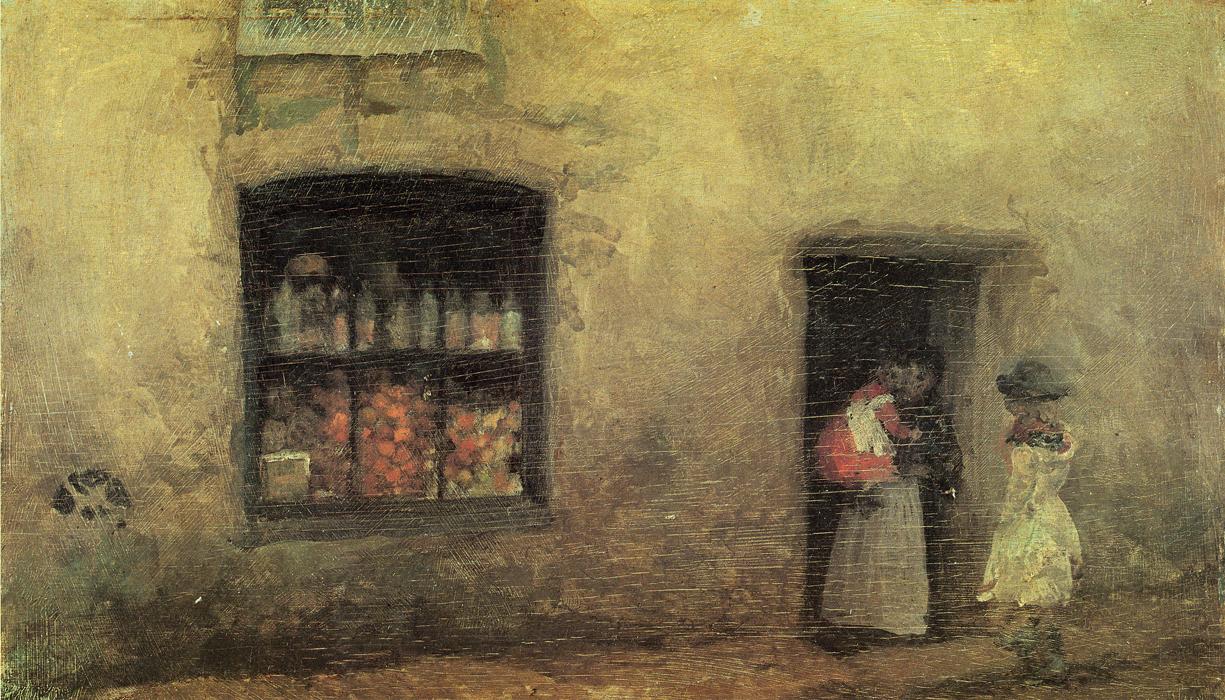This detailed painting depicts the facade of a rustic adobe-style building, featuring a tan and brown color palette that ranges from light to dark shades. The building's texture is accentuated with a mix of yellow and white wash, giving it a weathered look. On the left side, there is a window with neatly organized items inside, forming three rows of reddish and yellowish circular shapes at the bottom, resembling fruits, with bottles arranged on a shelf halfway up. The window has six panes of glass that offer a clear view of the contents inside.

To the right of the window, a scene unfolds at the entrance of the building. In the doorway, a woman dressed in a black top and a white apron holds a child, who is adorably dressed in a red and white outfit. Next to them, another young woman, clad in a knee-length white dress and a broad gray hat, is approaching. The ground in front of the building is a stone path with a slightly reddish tinge, contributing to the painting's nostalgic ambiance. This scene, reminiscent of a vintage marketplace, captures a moment of everyday life, possibly from a bygone era.